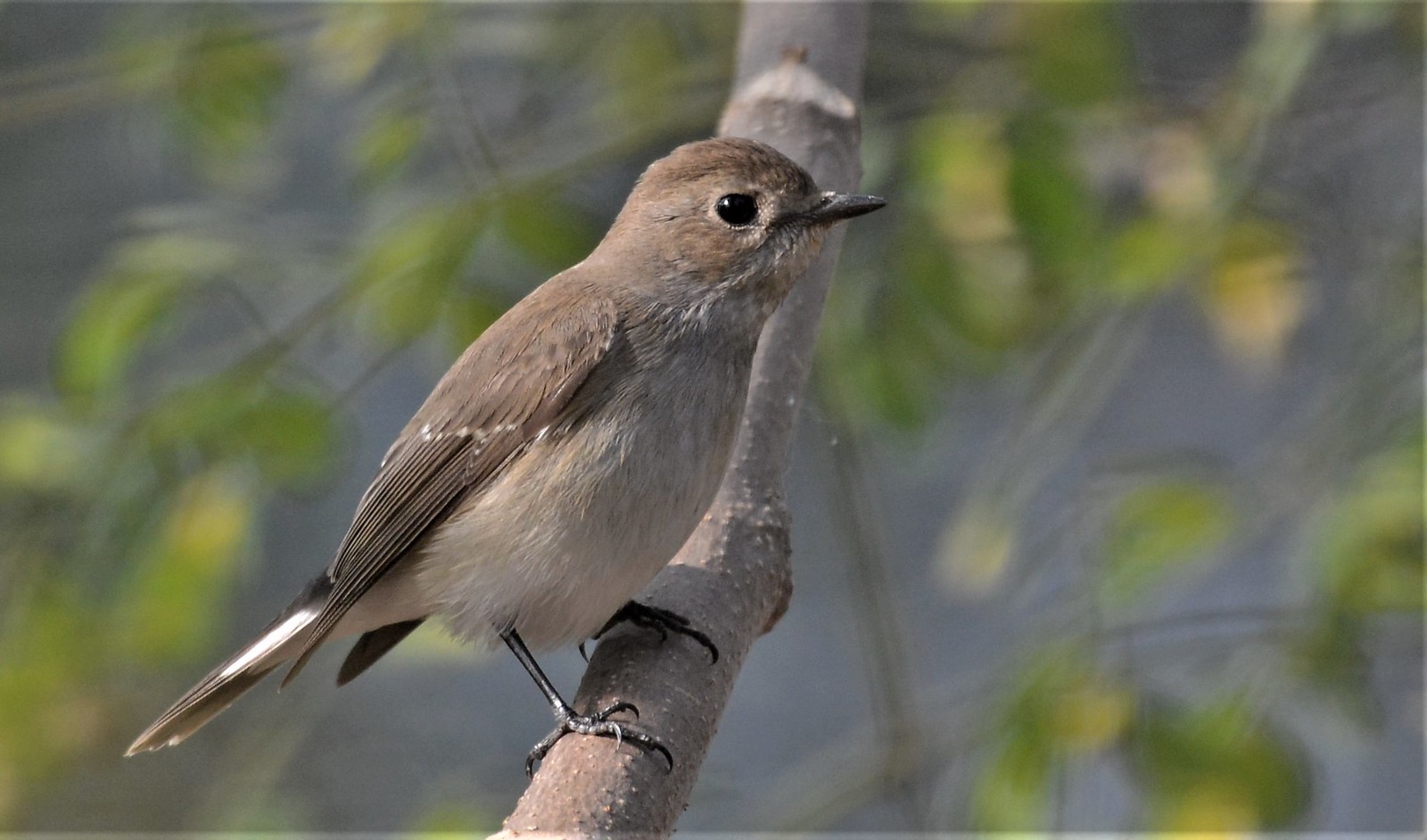This photograph captures a small bird, possibly a wren or a sparrow, perched gracefully on a tree branch. The bird's plumage is a harmonious blend of brown, beige, and tan, creating a subtle yet intricate pattern. It is posed in profile, giving a clear view of its small, pointed beak and distinct single black eye. Delicate white markings accentuate its tail feather and wings, adding a touch of contrast to its earthy tones. The surrounding branches are enveloped in lush green foliage, but the background is artistically blurred, ensuring the bird remains the central focus of this captivating image.